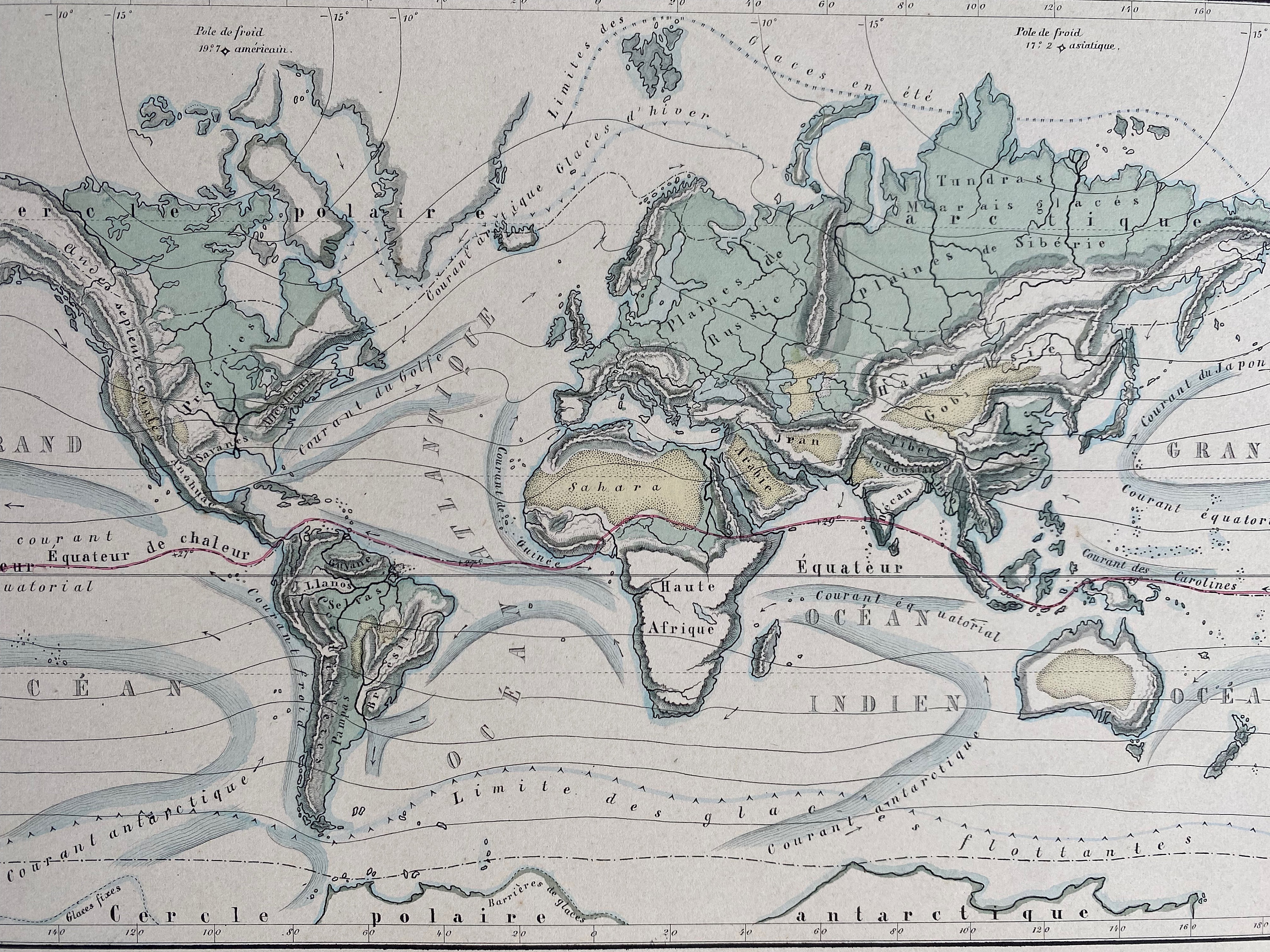The image showcases a detailed world map, primarily in green, brown, and gray colors. The continents – North America, South America, Europe, Asia, Africa, Australia, and Antarctica – are depicted without specific labels. Green signifies landmasses, while deserts like the Sahara in Africa are marked with red and brown colors. The map text is in French, with specific geographic features such as prairies in the United States, Sahara, Arabian Desert, Iranian deserts, and the Gobi Desert labeled. Oceans and significant geographical lines like the equator, Arctic Circle, and polar regions are clearly marked with thick and thin black lines. A red, wavy line traverses the map horizontally from left to right. At the bottom of the map, labeled 'Seco, Polar and Antarctic,' a black scale is present, and the image maintains a square format.